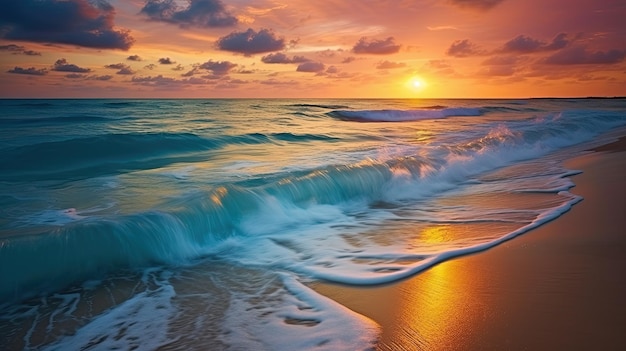This is a stunning computer-generated image of the ocean at sunset. The scene features a serene beach with smooth, satiny sand on the right side, casting a soft reflection of the setting sun. The sun, a glowing yellow orb, is positioned slightly right of center, illuminating the sky with rich shades of orange, honey, and amber. Large, puffy clouds punctuate the sky, appearing purple from underneath as they catch the fading light. The ocean itself is a mesmerizing pale turquoise that transitions to light blue, with gently rolling waves that create white foamy patches as they meet the shore. The waves, while dynamic, maintain a smooth appearance and the vivid reflections of the sun stretch in a straight line across the water, enhancing the tranquil beauty of the scene. The overall ambiance is peaceful and picturesque, capturing the quintessential elements of a coastal sunset.